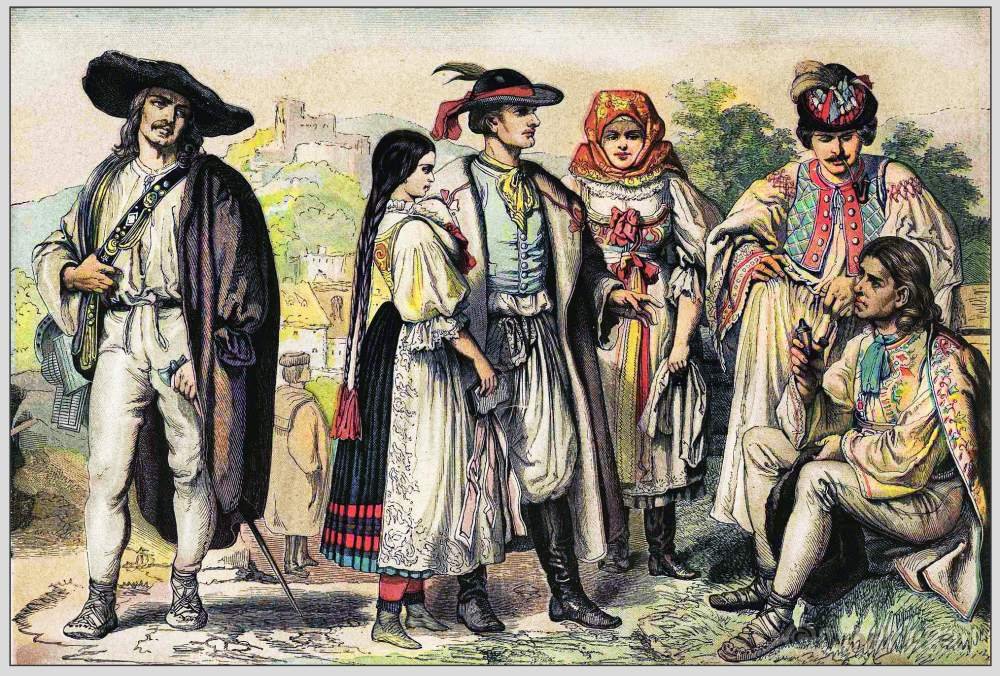The drawing depicts a scene from the 1700s featuring six individuals dressed in traditional Romanian folk costumes. On the far left, a man stands slightly apart from the group, holding a walking cane in his left hand and wearing a wide-brimmed black hat, an open robe, a white shirt, and pantaloons, with a swashbuck belt hanging from his shoulder. He has a goatee with a mustache and long dark hair. To his right is a group of five people gathered around a seated man who appears to be speaking. Among the group, two men and two women are attentively listening. The women are dressed in long skirts, one with a brown headscarf and one with long braided hair, while the men wear traditional bloomers, vests, and overcoats. The seated man, who is the focus of their attention, wears an elaborate shirt with gold details and white pants. In the background, a mountain with a castle on top can be seen, adding to the historical ambiance of the scene.